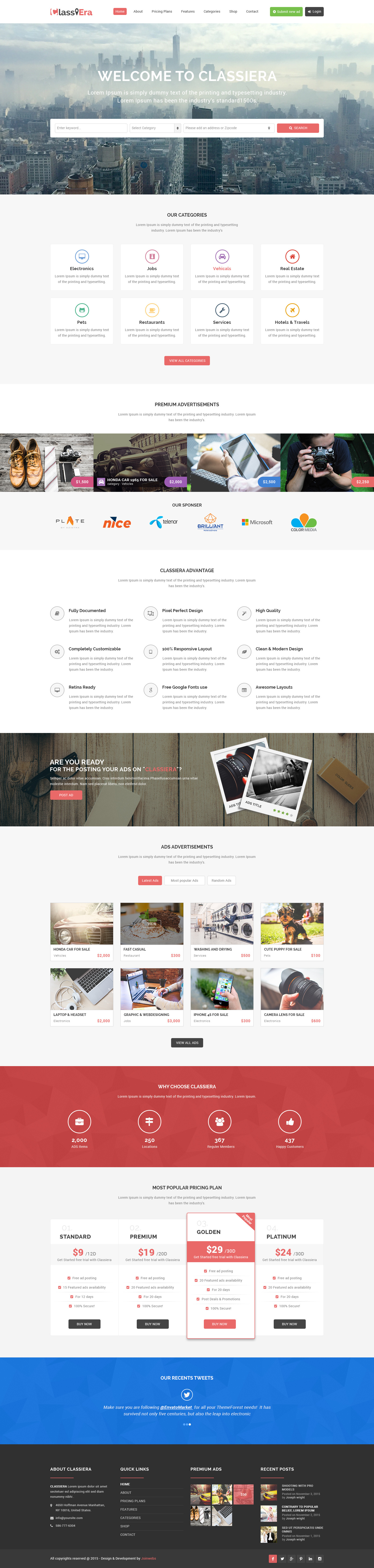Displayed here is the initial section of a basic website homepage. At the very top, the website features a narrow red bar, possibly containing text, with a smaller red segment adjacent to it. Positioned on the far right of the red bar are green and black elements.

Beneath this top section is a wide banner displaying an image of a city skyline, featuring the text "Welcome to Classiva" superimposed on it. Below this city image, there's an elongated search bar spanning the width of the website.

Following the search bar, a section with eight interactive options is presented, arranged in a grid formation with four options per row and two rows in total. Below this grid, there is a bar containing pictures, leading to additional selections.

Further down, another set of interactive choices is displayed, followed by another picture bar. Continuing the layout, there are smaller images again arranged in a four-by-two format.

The lower part of the site features a series of color-coded bars: a red bar with four choices, followed by a blue bar, and then a black bar.